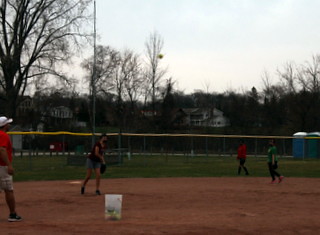In this small, low-quality image of a baseball field, there are four people casually playing what looks like a pickup game, evidenced by their varied outfits, including shorts and T-shirts without any formal gear. A man near the pitcher's mound is wearing shorts and a red baseball cap. Surrounding the dirt pitcher's mound is well-cut green grass, encased by a greenish fence. A distinctly visible bucket with a red handle sits on the field, partially filled with green items. The backdrop features leafless tall trees, suggesting it might be winter, alongside two white houses and a flagpole. In the distance, port-a-potties are visible, adding to the informal setting. The overcast sky gives a white hue, enveloping the scene in a muted light.